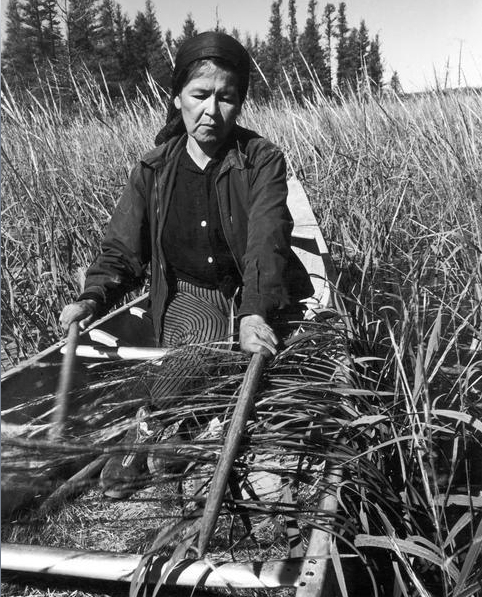This black-and-white photograph captures an older woman, possibly of East Asian, Native American, or Hispanic descent, sitting in a canoe-like vessel amidst a field of tall grass or wheat. She has darker skin and a serious expression. The woman is dressed in a black shirt covered by a dark jacket with white buttons, and she wears striped trousers. Her head is wrapped in a black scarf. She holds two sticks or oars in her hands, suggesting she might be propelling or steering the vessel. Despite the canoe shape, there's no visible water, indicating that the boat might be used for agricultural purposes. The background features tall pine trees under a gray sky.